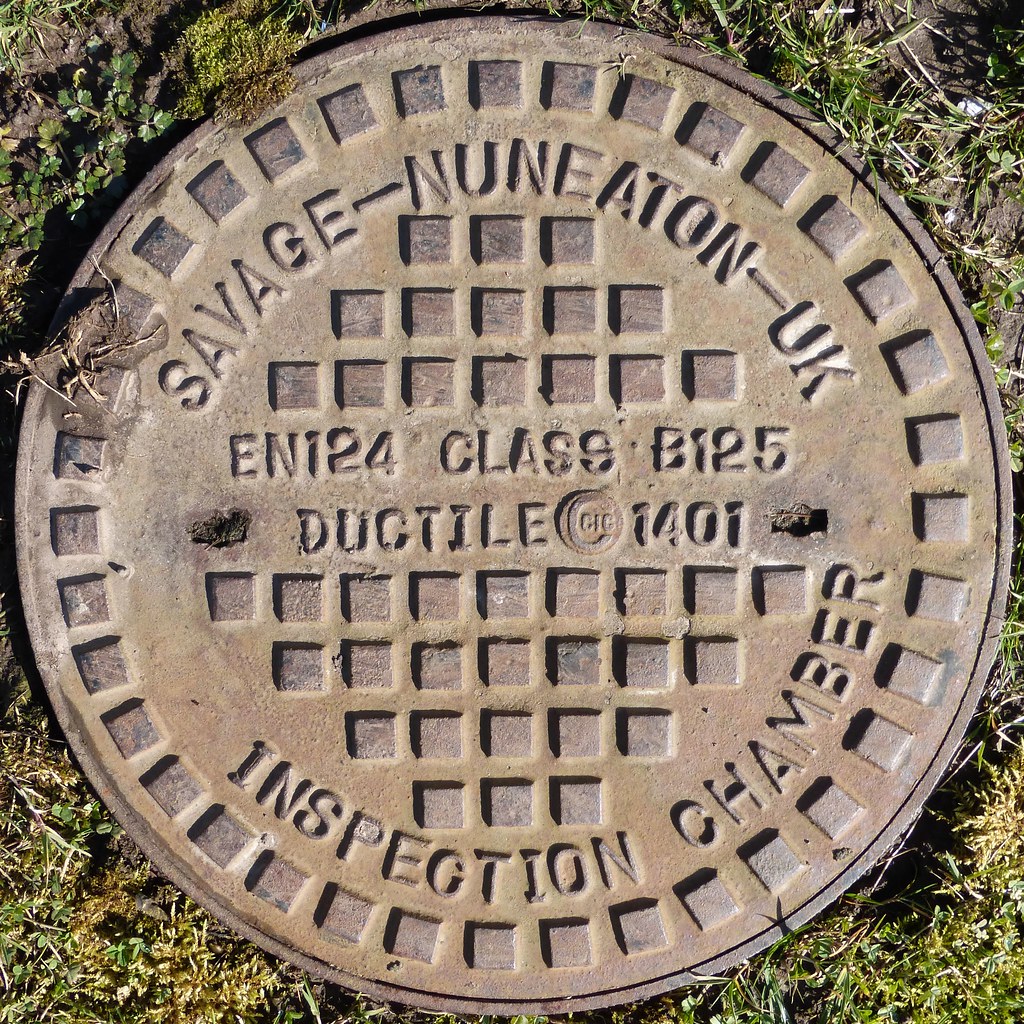The image depicts a heavy, circular metal object, likely a sewer cover or manhole cover, set amidst a grassy area. The cover is made of a dark, grayish-brown material, suggesting it's crafted from steel or ductile iron. Prominently featured on its surface is an arrangement of text: "SAVAGE NUNEATON UK," "EN124 CLASS B125," "DUCTILE 1401," and "INSPECTION CHAMBER." The design of the cover includes a pattern of squares spread across its face, enhancing its rugged appearance. The surrounding grass is primarily green with tinges of brown, framing the utilitarian yet sturdy cover.